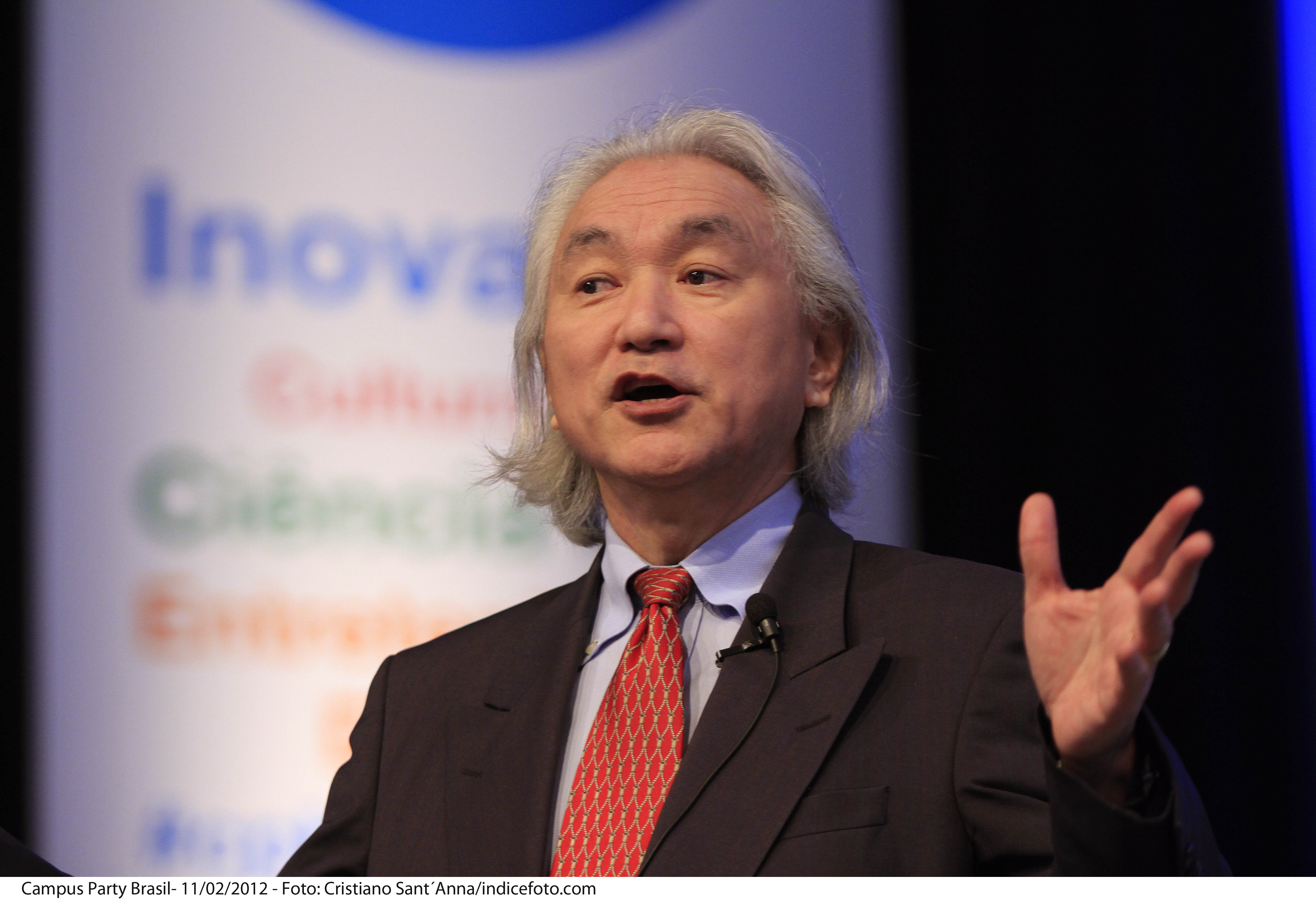This photograph captures an elderly Asian man with medium-length, straight gray hair, who is speaking on stage at what appears to be a conference or presentation. He is gesturing with his left hand raised. He is dressed in a dark gray suit jacket with a light blue shirt, and a red tie featuring a crisscross or diamond pattern. A small microphone is attached to the left lapel of his jacket. Behind him, a sign partially reads "INOVA" with additional red, green, and orange letters beneath, though they are too blurred to be legible. The caption at the bottom of the image reads "Campus Party Brazil 11-2012, photo Cristiano St. Anna / indicephoto.com."